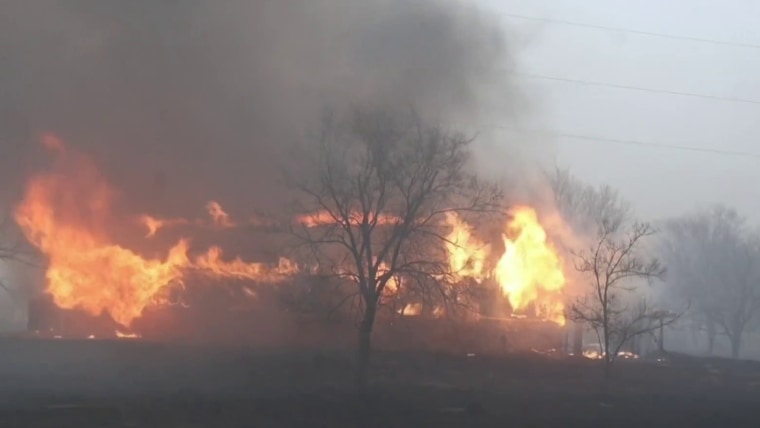The image depicts a large and severe structure fire engulfing a substantial building, with bright orange and yellow flames prominently emanating from the left middle of the structure and rising vigorously into the sky. The fire appears to be completely out of control, enveloping the entirety of the building and producing thick, heavy black and gray smoke that dominates the left side and middle of the image. The smoke is so dense that it obscures parts of the scene, contributing to the overall chaotic and somber atmosphere. In the foreground, there are several bare trees without leaves, suggesting either seasonal bareness or damage from the fire. These trees are situated in the front middle and to the right bottom of the image. Additionally, three power lines stretch across the upper portion of the image, though they become less visible toward the left side due to the heavy smoke. The ground in front of the structure is dark and indistinct, adding to the overall bleakness of the scene.